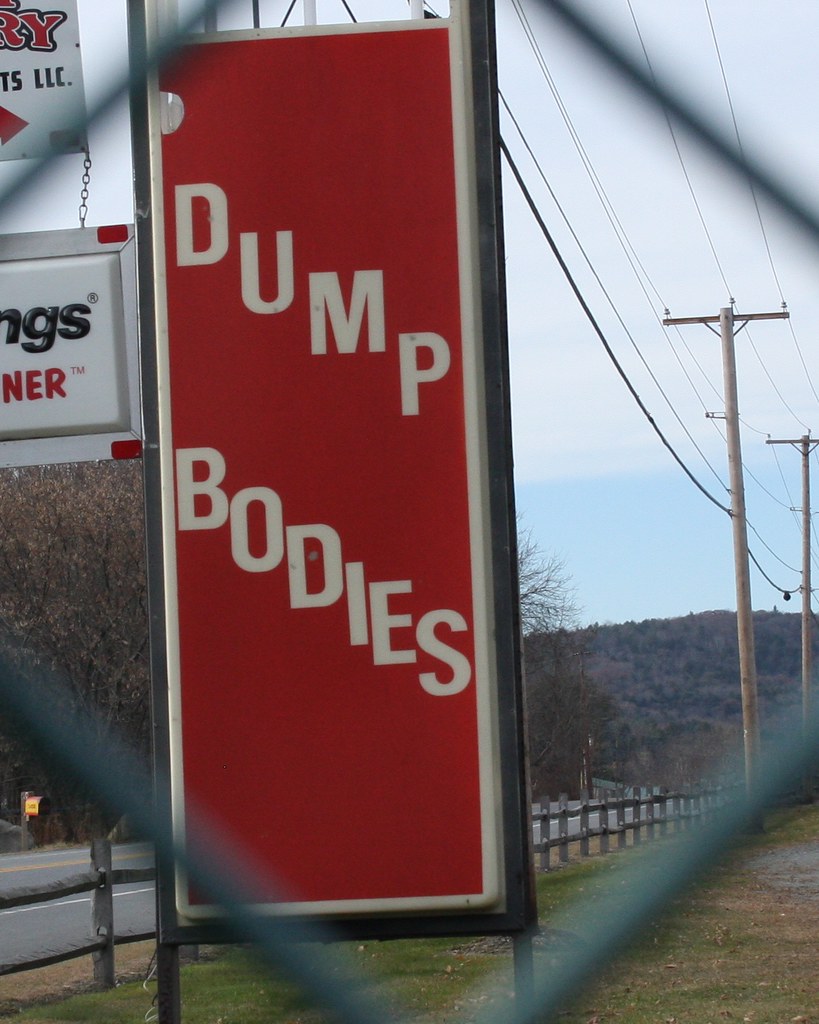The image is captured from behind a chain-link fence and shows a close-up of a large rectangular sign next to a country road. The prominent red sign has white letters that read "dump bodies," with the words arranged diagonally. The road is visible to the left and runs horizontally across the image. A wooden fence lies between the road and the sign. In the background, there are hills covered with trees and brown grass, indicating a fall setting, as well as some bare trees and a large tree with brown leaves to the left of the road. Additionally, there are multiple electric poles with power lines running alongside the road. Another white sign, partially visible and possibly made of paper, appears to be chained together with the main sign. The surroundings are green with patches of grass under the sign.